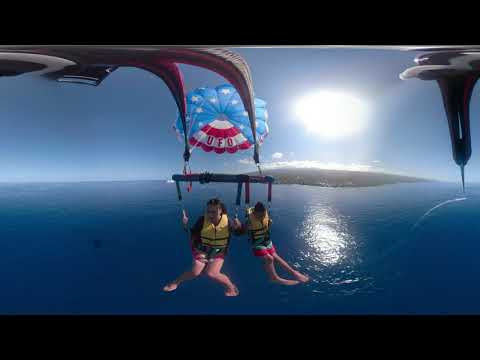The photograph captures a dramatic fisheye perspective of two Caucasian individuals, possibly kids, parasailing over a dark ocean under a blazing sun. They are strapped into a harness system, suspended from a thick bar, and holding onto the harness's straps, which secure them to a colorful parachute billowing behind. They are both dressed in red shorts and yellow life preservers. The parachute, embellished with stars and stripes of the American flag motifs, features a prominent white stripe with the red letters "UFO" emblazoned on it. In the surrounding scene, the sky appears slightly blurred, hinting at the intense sunlight. An island is visible in the distant background, while the water below shimmers with the sun's reflection. On the right edge of the image, another unidentified pointed object is faintly visible, adding to the complexity of the composition.